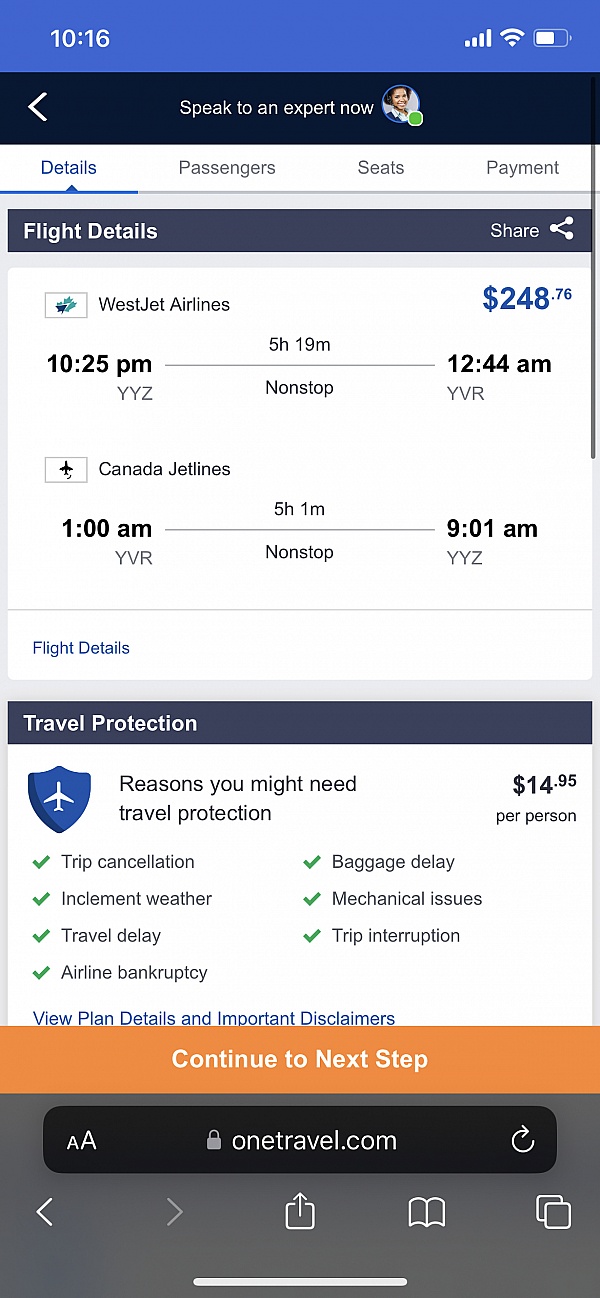The image depicts a smartphone screen displaying a travel booking website. The current time on the phone is 10:16, though it is unclear whether it is AM or PM. The Wi-Fi signal is active, and the battery is approximately two-thirds full. 

At the top of the screen, there's a black bar below a blue header. This black bar features the text "Speak to an expert now" in white, accompanied by a chat button. Below this is a white navigation bar with sections labeled "Details," "Passengers," "Seats," and "Payments," with the "Details" section highlighted.

The detailed flight information follows:

- **Outbound Flight:**
  - **Airline:** WestJet Airlines
  - **Price:** $248.76
  - **Departure:** 10:25 PM from YYZ (Toronto Pearson International Airport)
  - **Arrival:** 12:44 AM at YVR (Vancouver International Airport)
  - **Flight Type:** Non-stop

- **Return Flight:**
  - **Airline:** Canada Jet Lines
  - **Departure:** 1:00 AM from YVR
  - **Arrival:** 9:01 AM at YYZ
  - **Flight Type:** Non-stop

Below the flight information, there's a section on travel protection with the heading "Reasons you might need travel protection," citing reasons such as trip cancellation, inclement weather, and travel delay. The cost for travel protection is listed as $14.99.